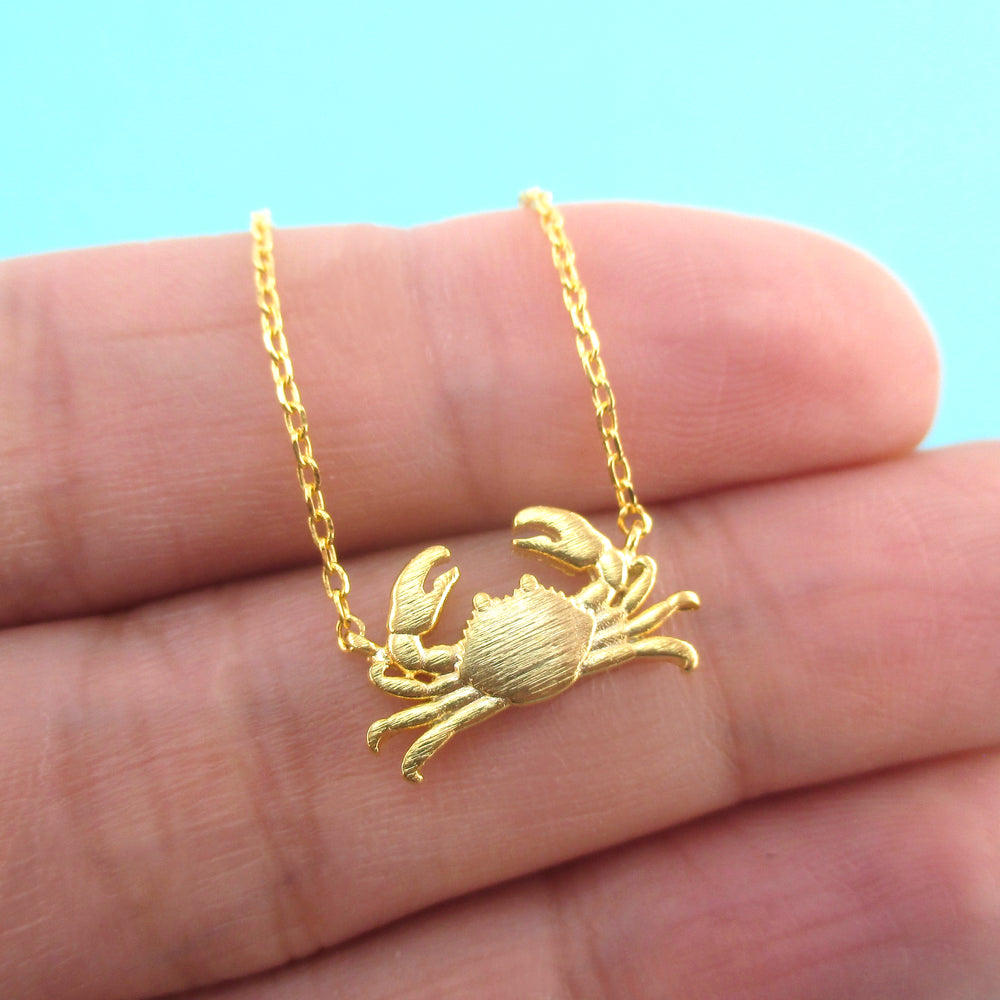This vertical close-up image focuses on a person's hand, difficult to identify as male or female, with notably large fingers. The hand is holding a delicate gold necklace featuring a crab charm. The intricate detailing of the crab is clear, showing its body, legs splayed in different directions, and claws raised above. The necklace drapes elegantly over three prominent fingers – the index finger holding the chain, the crab charm resting on the middle finger between the first and second knuckles, and part of the ring finger is visible too. The background is a solid turquoise or sky-blue color, which contrasts sharply, making the gold of the necklace and the detail of the charm stand out. The crab charm appears quite small, probably smaller than a penny, emphasizing the closeness of the shot and the delicate craftsmanship of the jewelry.